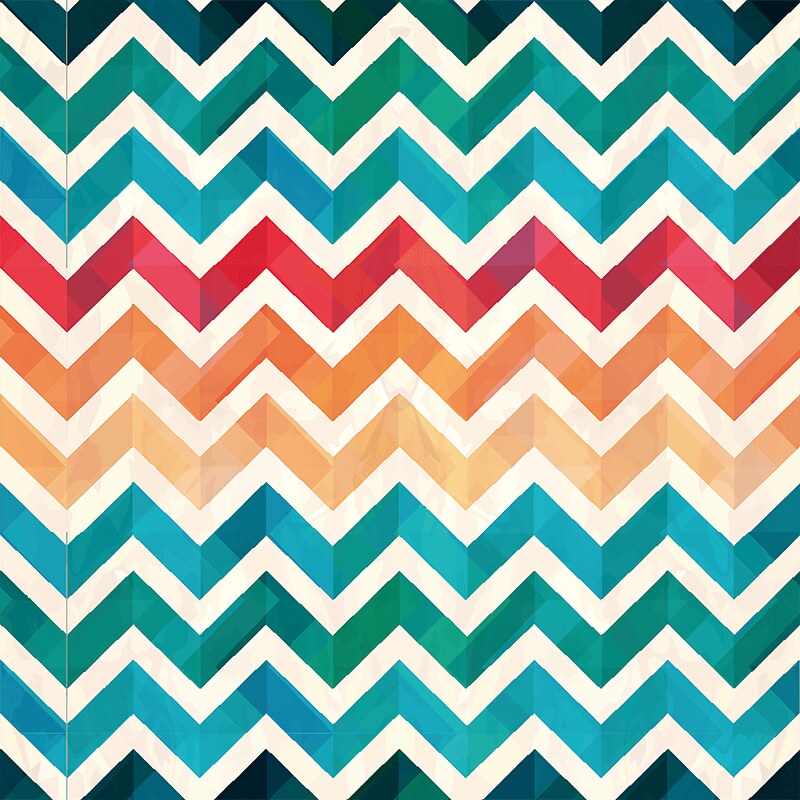The image depicts a perfectly square pattern of chevron design lines, characterized by a series of jagged, squiggly lines in various colors, with white spaces in between each line enhancing the chevron appearance. The design begins at the top with dark green transitioning to lighter greens, followed by a sequence of blues, red, orange, yellow, and then repeating blue below the yellow. The middle section prominently features red, orange, and yellow hues. Further down, the sequence resumes with teal, varying shades of green, and dark green, culminating in teal again at the bottom. Overall, the dominant colors—green, blue, red, orange, and yellow—are symmetrically echoed from the top to the bottom of the pattern, with the teal and green colors appearing more frequently.